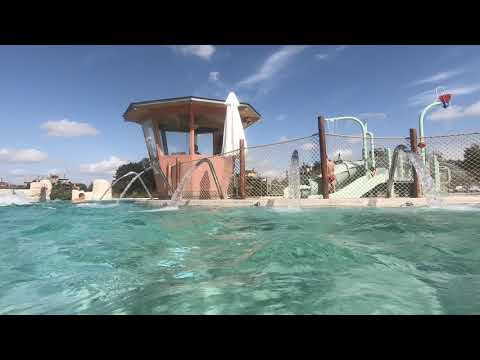The image depicts a recreational swimming pool filled with clear blue water, allowing an unobstructed view to the bottom. Edging the pool are multiple wooden fence posts intertwined with brown netting, serving as a barrier. Three bent spouts shoot arcs of water back into the pool. Dominating the center of the image is a peach-colored octagonal structure with multiple windows on each wall and a flat roof. Adjacent to this structure is a folded outdoor umbrella. Behind the fence is a light blue slide and more wooden poles visible in the distance. The sky above is a light blue adorned with fluffy white clouds. On closer examination, a male swimmer's head can be seen at the far left edge of the pool. The scene is vibrant yet serene, capturing a peaceful day at the pool.